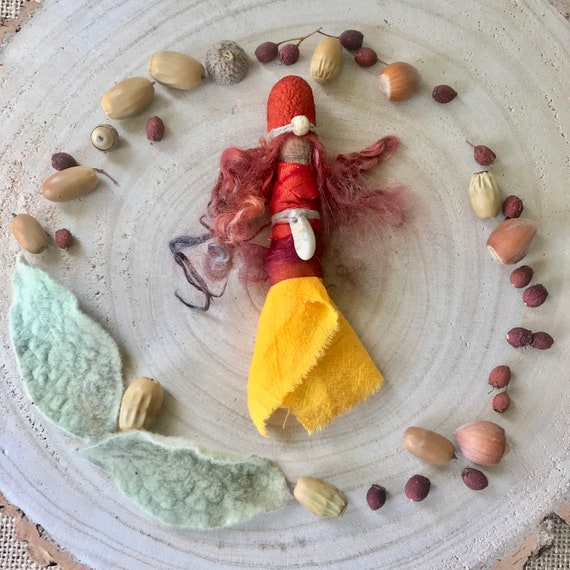The image captures a meticulously arranged scene on a white lace background, possibly taken outdoors given the bright lighting. Central to the composition is a handmade doll made from a cork, adorned with reddish-burgundy hair and wearing a red outfit that transitions into a yellow felt skirt. The doll has no face but features a felt hat with a white bead in the center. Surrounding this doll is a symmetrical circle of various natural elements like acorns, seeds, and nuts, which vary in color from beige to brown and even burgundy. Two dried felt leaves are placed within the circle, enhancing the artistic and possibly ritualistic feel of the display. This arrangement of nature and craft materials creates a striking, almost ceremonial focus on the doll in the middle.